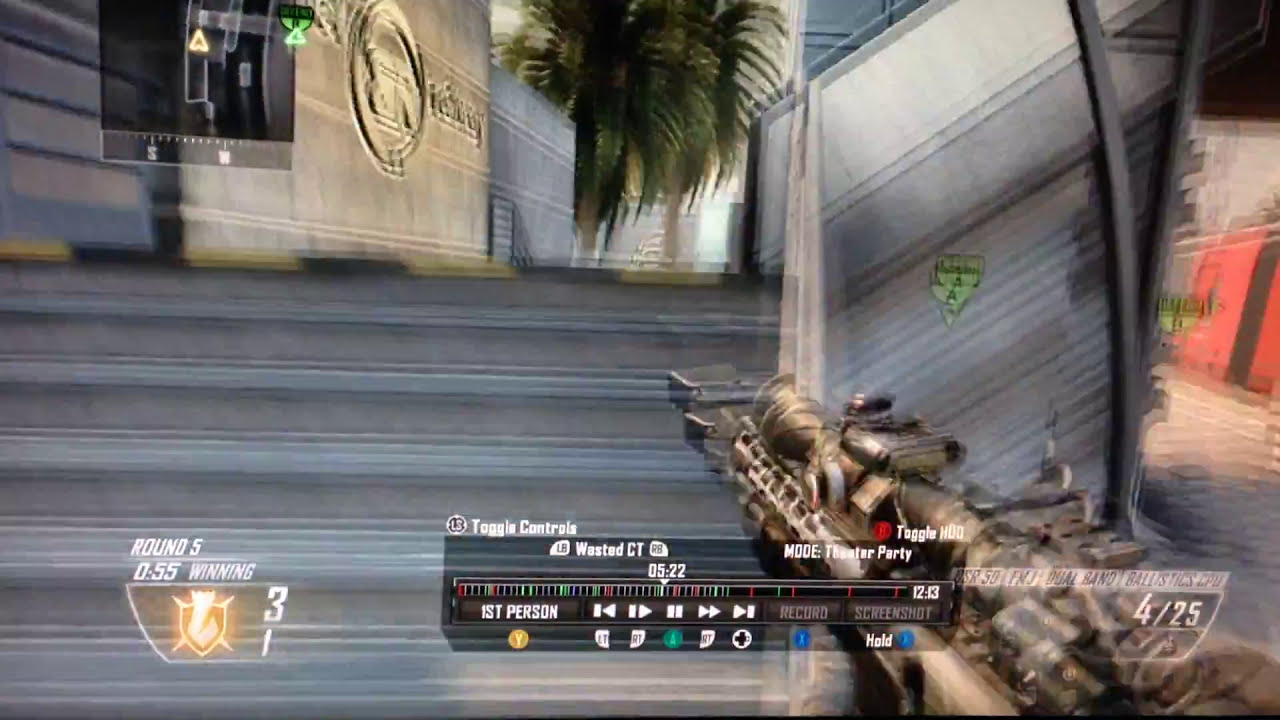The image is a blurry screenshot from a first-person shooter video game, featuring a high-tech automatic weapon held in the bottom right corner. The player appears to be navigating a staircase that starts on the left and turns to the right, extending out of the frame into the top right corner. The setting of the game seems to be in a war environment, indicated by the staircase built within a building and a visible palm tree. At the bottom left, the screen displays "Round 5," a timer set at 55 seconds, and a message "Winning." Accompanying these are icons, including a shield with the numbers "3/1" and various game controls and buttons. The top left corner features a mini-map and a gold emblem with a black box containing a yellow triangle. The bottom center includes a video track interface that allows for fast-forwarding and pausing. Prominent colors in the image include shades of gray, white, yellow, green, blue, red, and gold, contributing to the chaotic and intense atmosphere of the game.